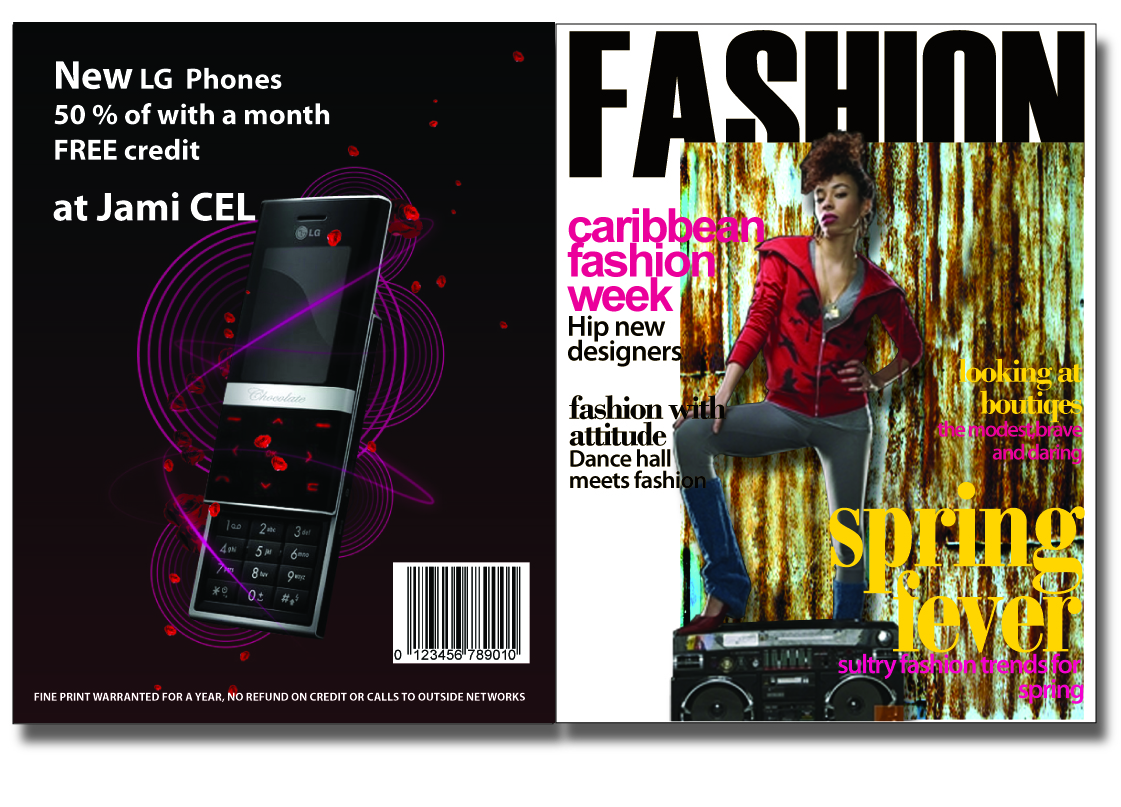The image showcases both the front and back covers of a magazine side by side. The back cover, positioned on the left, features a black advertisement for new LG phones. The ad highlights a promotional offer: "50% off with a month free credit at JamiSell." It includes a picture of a classic black LG slide-up phone set against a background of intertwining red-violet and purple circles, and a barcode is located at the bottom right. Small white text at the bottom states, "Warranted for a year; no refund on credit or cost to outside networks."

The front cover on the right is predominantly white with the word "Fashion" in bold black font at the top, slightly obscured by a central photograph of an African American woman. She has large brunette hair styled voluminously at the front and shorter at the back. Dressed in a red zip-up jacket over a large V-neck grey shirt, gray pants, and boots or heels, she stands confidently with one foot on an old black boombox. The background features a rust-colored wall with white accents. Surrounding the model, various headings promote magazine contents in vibrant colors: "Caribbean Fashion Week," "Hip New Designers," "Fashion with Attitude," "Dance Hall Meets Fashion," "Spring Fever," "Sultry Fashion Trends for Spring," and "Looking at Boutiques: The Modest, Brave, and Daring."